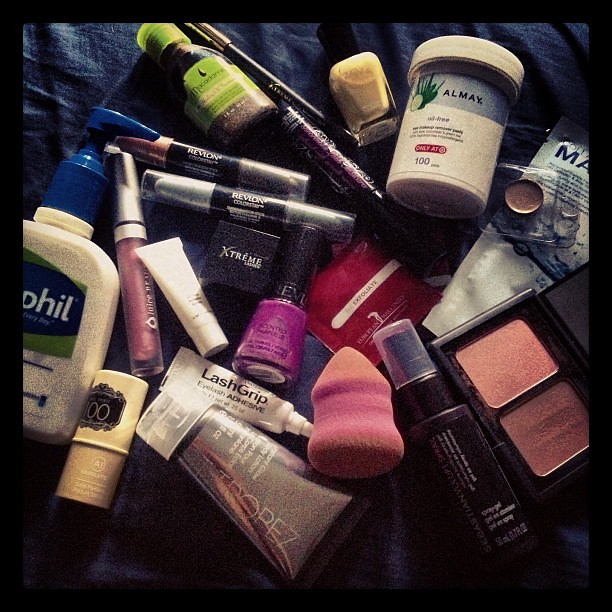The image showcases an assortment of beauty products artfully arranged on a slightly wrinkled, dark blue cloth. At the top center of the image, there is a bottle flanked by two tubes, all unlabelled. Moving rightward, a container reminiscent of a pill bottle displays the "Almay" brand. Adjacent to this is a Cetaphil container equipped with a pump. Further right, two Revlon tubes, likely lipsticks, stand next to a vertically aligned, unidentified tube. Below this, a bottle of nail polish catches the eye with its vibrant purple hue and contrasting black lid.

To the left, a square container in bold red sits mysteriously, its contents unknown. A pale yellow object, possibly a beauty product, can be seen nearby, along with an unlabeled tube. Above, the words "Lash Grip Adhesive" are discernible on another product. Rightward, a spongy applicator, probably for smoothing out powder, lies next to a spray bottle.

Completing the display is a compact featuring two shades of blush—one a lighter pink and the other a darker pink. The entire collection is showcased on a slightly rumpled dark blue cloth, adding a touch of casual elegance to the presentation.